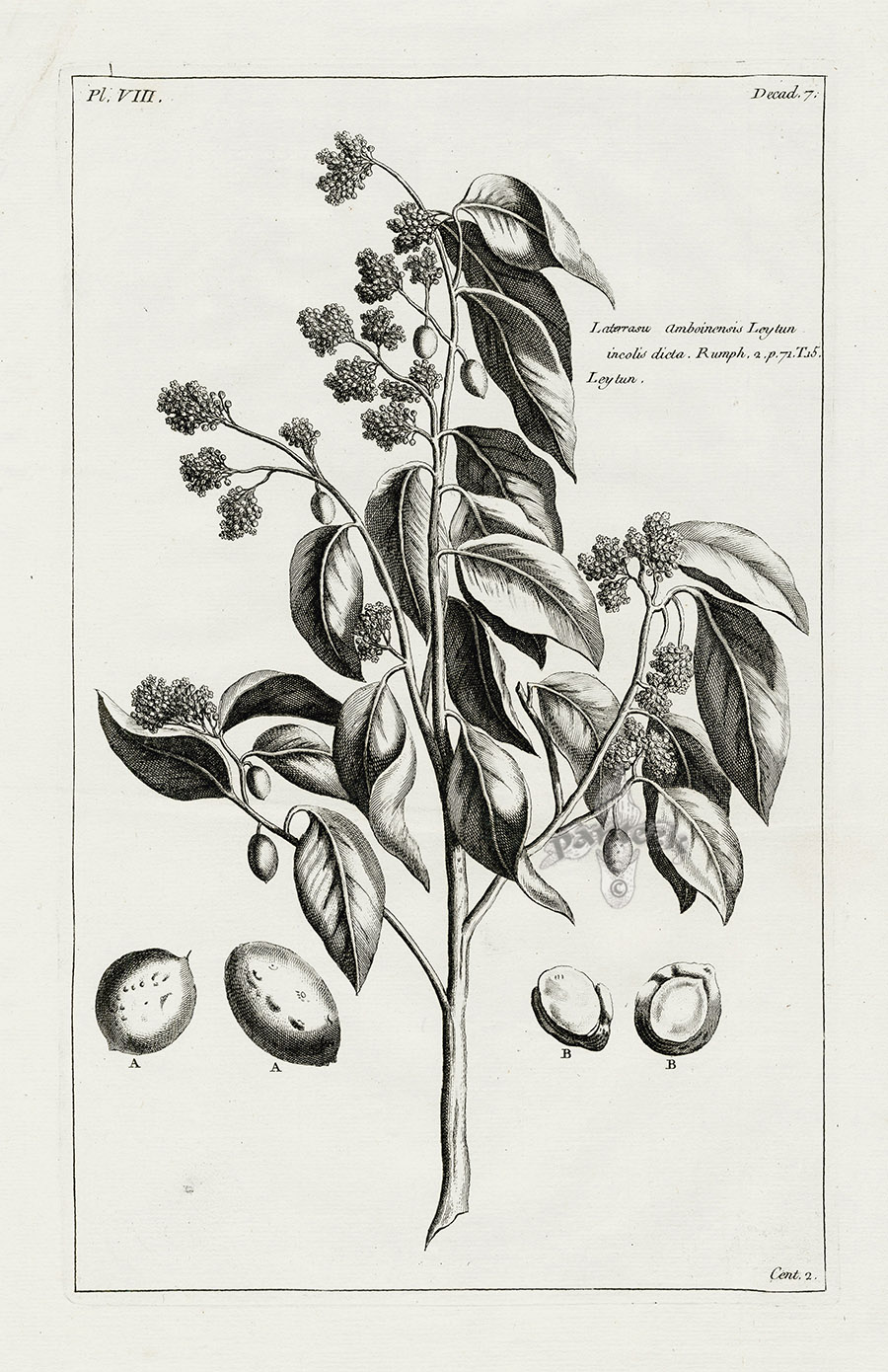The image is a detailed black and white pencil drawing of a plant, possibly sourced from a flora and fauna textbook and aligned vertically on white paper. The scientific notation at the top, which is difficult to decipher but seems to read 'Labtran something,' identifies the plant. The plant features a wooden-looking stem with leaves, and towards the top, it has berry-like fruits. At the bottom left, two fruit-like structures are depicted, while at the bottom right, two circular objects marked 'A' and 'B' illustrate additional details. The plant has flowers at the tips of its branching stems. A text blurb at the top right provides more identification details about the plant.